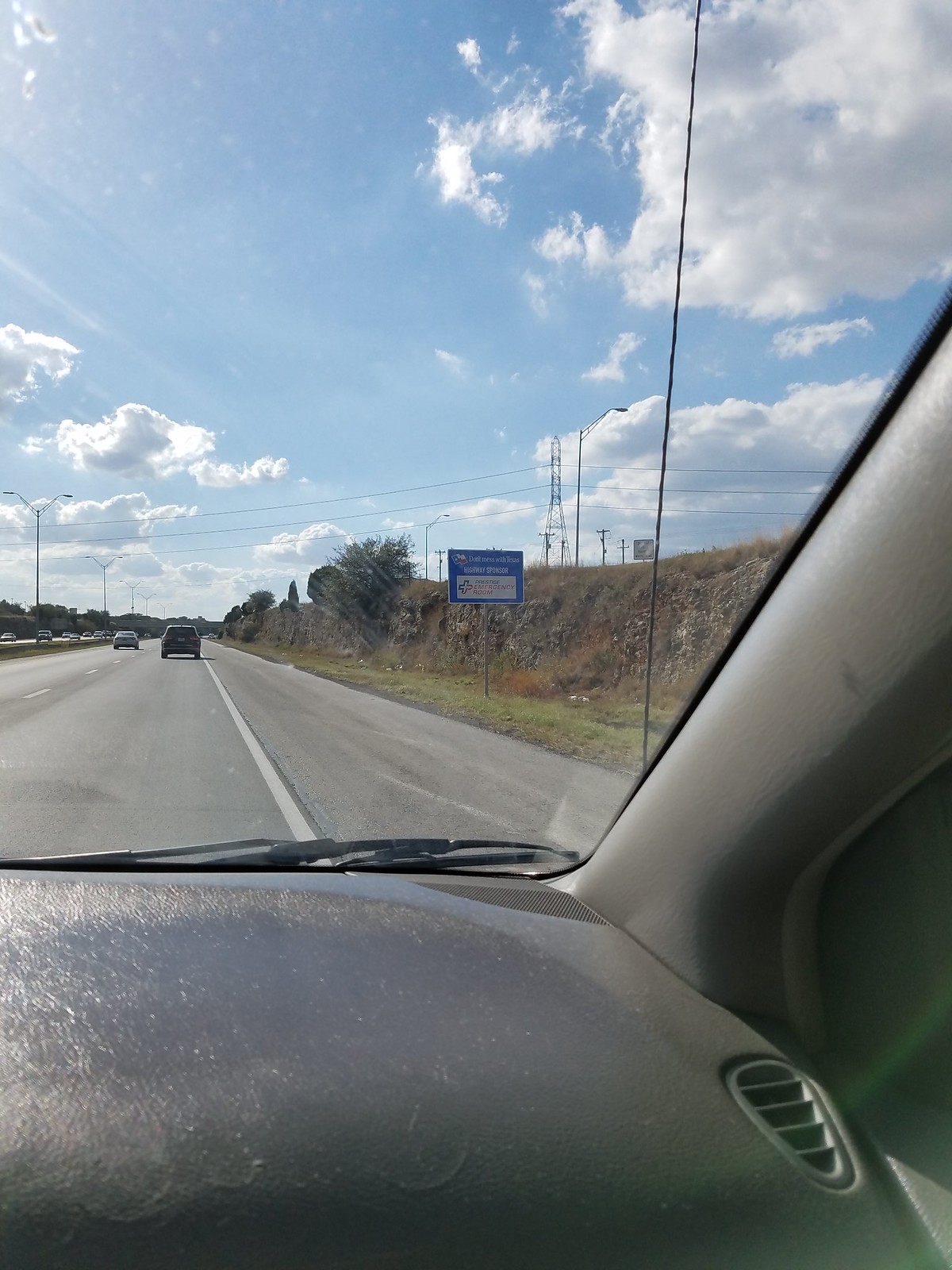This photograph captures the view from inside a moving car on a sunny day with clear, blue skies and puffy white clouds. Taken from the passenger side, the image shows the shiny, armor-walled dashboard, which is either gray or black, featuring a window vent, a speaker grill, and the arm of the windshield wiper. Through the window, an expansive highway unfolds, bordered by grassy hills on the right and electrical grid lines stretching overhead. The car travels in the extreme right lane of a four-lane highway with oncoming traffic visible on the opposite side. Ahead, there is minimal traffic with a few car lengths between vehicles, allowing a clear view of a blue information sign indicating an emergency room. A black antenna and the gray post of the sign are also noticeable, along with a distant tower on the right side of the image.